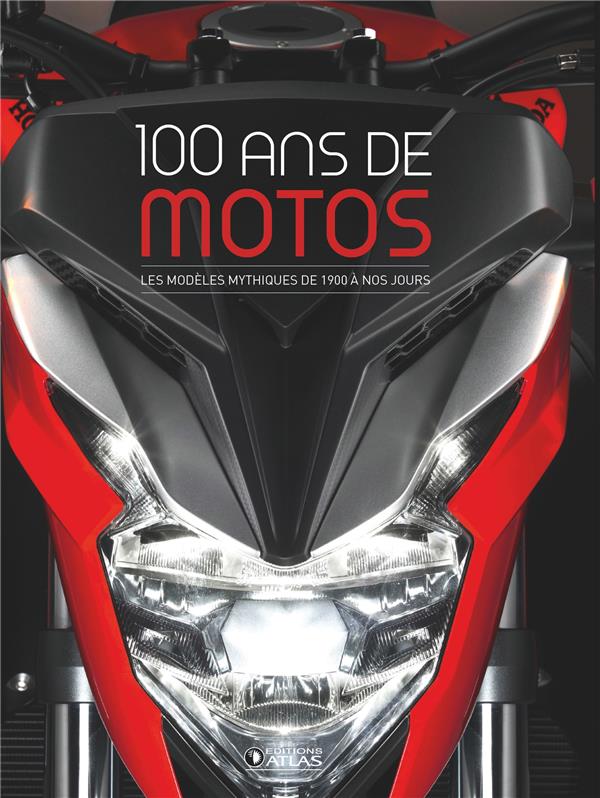This image is a detailed color advertisement, likely from a magazine, showcasing the front view of a Honda motorcycle with a design that celebrates 100 years of motorcycle history, specifically from 1900 to 2000. The motorcycle stands prominently with a head-on perspective highlighting its black, red, and silver components. The cowl features the headlight in the middle, flanked by silver posts and partially visible black handlebars. A silver speedometer crowns the top, while the tank and the seat are painted red and black, respectively. This is complemented by a shiny light at the back and reflective elements by the footrests. The background is stark black, making the motorcycle and the text more striking. The text across the top reads in white "100 ANS DE" and in red "MODOS," followed by a smaller text beneath, which translates to "The Mythical Model of 1900," all in French, reinforcing the centennial celebration of motorcycle heritage.